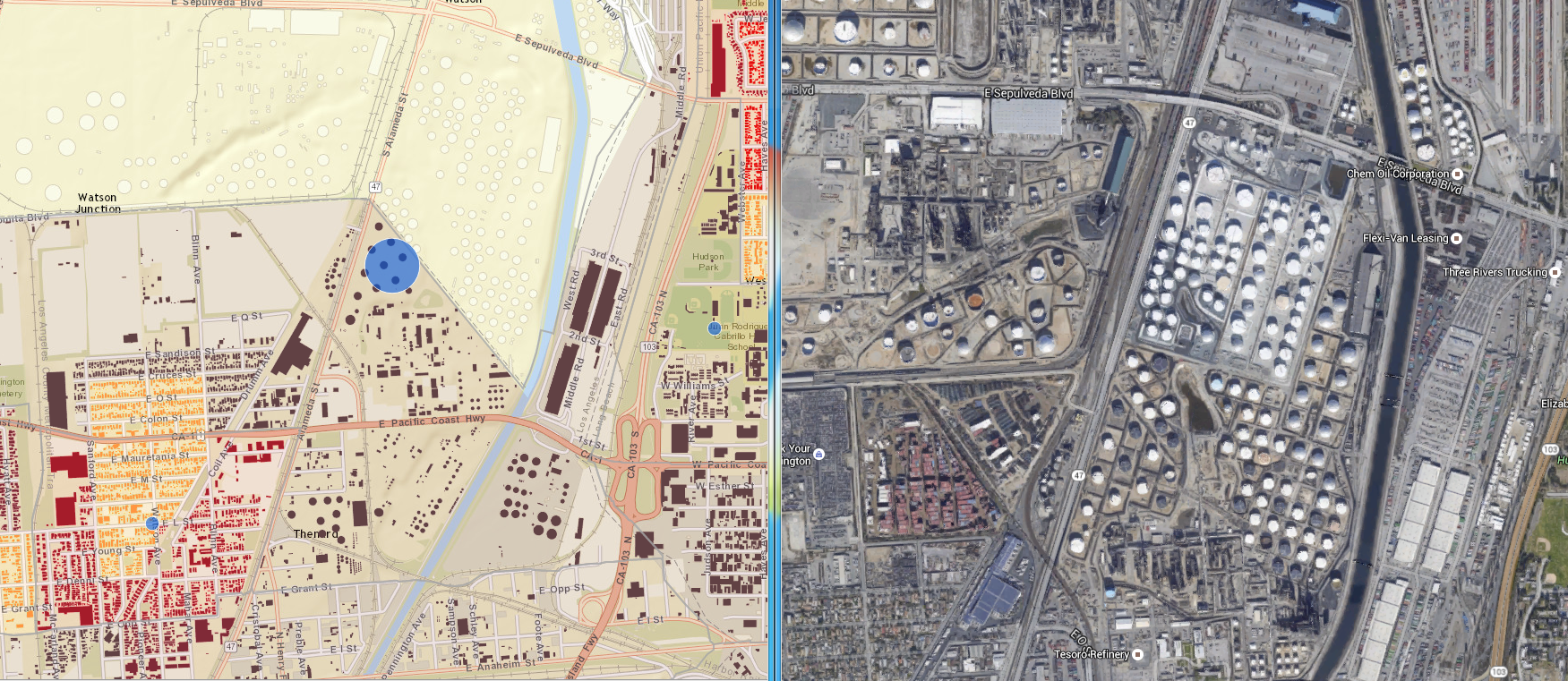The image on the right depicts a portion of a city map rendered in blues and grays. This map lacks any noticeable water features. Prominent features include two primary vertical roads: one on the right rendered in black, and another in the center rendered in gray. Additionally, a main road runs horizontally across the top before curving gently downwards at a slight diagonal to the right. Various sections of the city are indicated; one section is rectangular and filled with numerous white circles, though its purpose is unclear. Similar white circles are scattered throughout other areas of the map, albeit less densely. A section featuring reddish buildings also stands out, but its significance is difficult to interpret. Although there is writing on the map, it is illegible.

The image on the left is a contrasting city map in tans, oranges, reds, pinks, and some light green. Unlike the right-side map, this one appears to use an Asian script or perhaps another intricate symbol system that is difficult to discern due to its small size. The top sections of the map are ivory with small circles scattered throughout. Below these sections, the map transitions to a darker tan with segments of red and gold, creating a complex and somewhat confounding visual layout. Overall, the intent and specifics of this left-side map remain unclear.